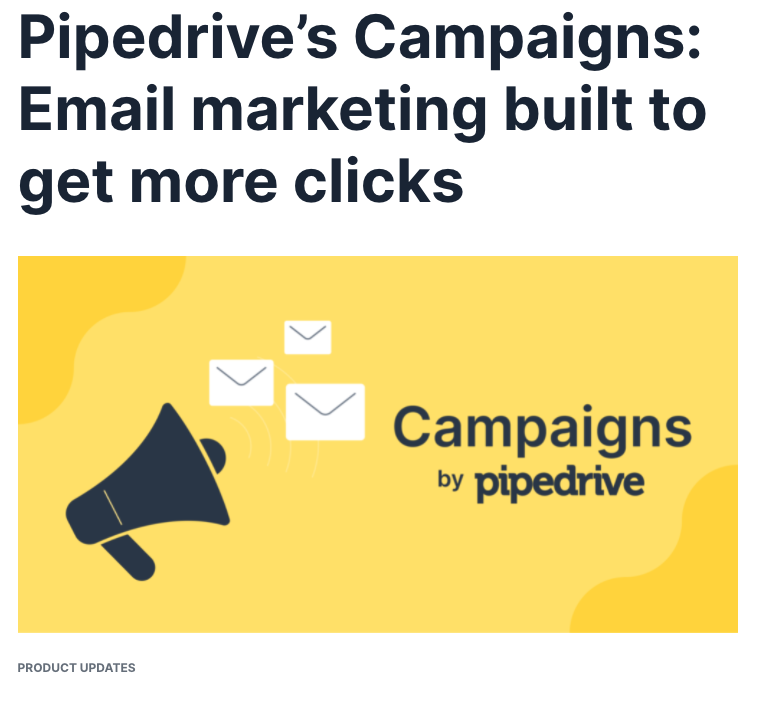The image features a white header area with the black text, "Pipedrive's Campaigns: Email Marketing Built to Get More Clicks." Below this, there is a rectangular shape with a gradient of two different tones of orange—darker in the top left corner and bottom right corner, while the center features a lighter orange separated by two wavy lines. On the left side of the orange rectangle, there is a black silhouette of a megaphone with three white envelopes floating in front of it. To the right of the megaphone, the word "Campaign" is displayed in large black text, followed by the word "by" in very small letters, and then "Pipedrive" in a slightly larger font size than "by," but smaller than "Campaign." Below the orange rectangle, there is another white area where "Product Updates" is prominently written in capital black letters on the left side.